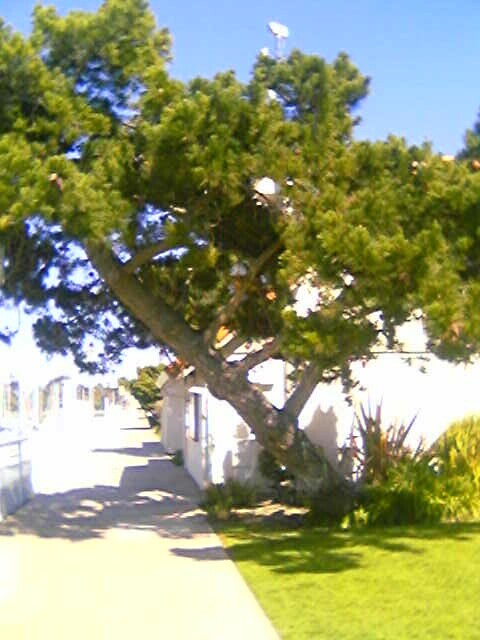The blurry photograph depicts a serene outdoor setting on a bright, cloudless day, dominated by a large, leafy tree growing at an angle. This tree, with its brown trunk and multiple branches, extends from the bottom right corner diagonally towards the top left, casting intricate shadows on the landscape below. To the right in the foreground, a meticulously maintained short-cut green lawn is bathed in sunlight and shaded patches. Adjacent to the lawn, a grey concrete sidewalk stretches far into the distance, lined with additional bushes and shrubbery that add to the lush ambiance. Partially obscured by the tree's foliage, a white house with a single visible window stands behind this natural tableau. The bright blue sky overhead illuminates the entire scene, casting shadows from the surrounding buildings, creating a picturesque and peaceful atmosphere.